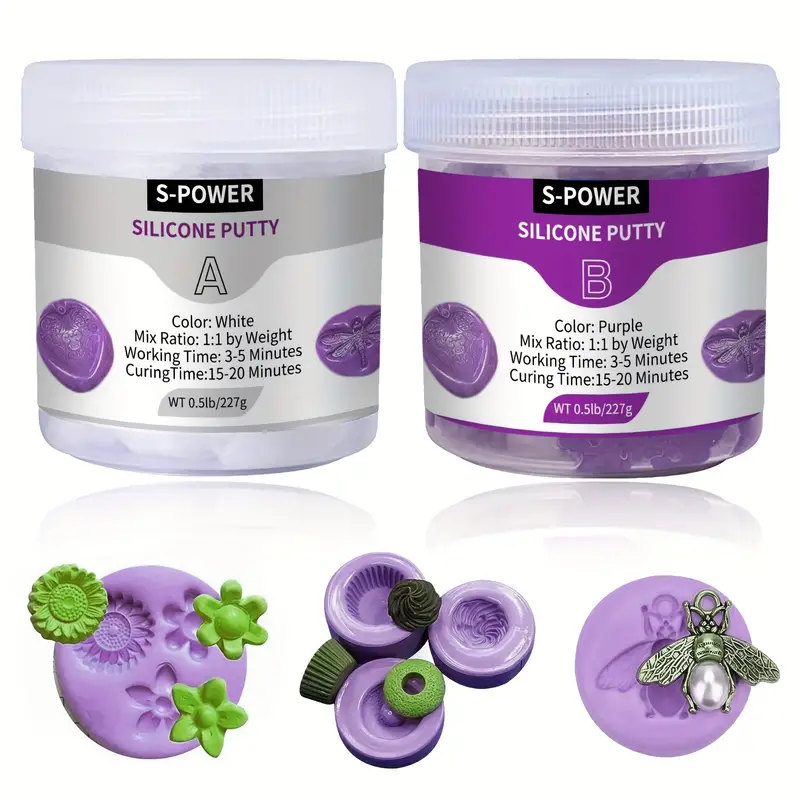The image features two identical containers of S-Power Silicone Putty, each with distinct color labels. The container on the left has a gray background and contains white putty, labeled as "Silicone Putty A." The container on the right, with a purple background, holds purple putty and is labeled "Silicone Putty B." Both containers specify a mix ratio of 1 to 1 by weight, with a working time of 3 to 5 minutes and a curing time of 15 to 20 minutes. Additionally, they each weigh 0.5 pounds or 227 grams. At the bottom of the image, there are examples demonstrating the putty's use, showcasing various imprints and shapes, including circles, flowers, and other objects, suggesting a range of creative applications for arts and crafts projects.